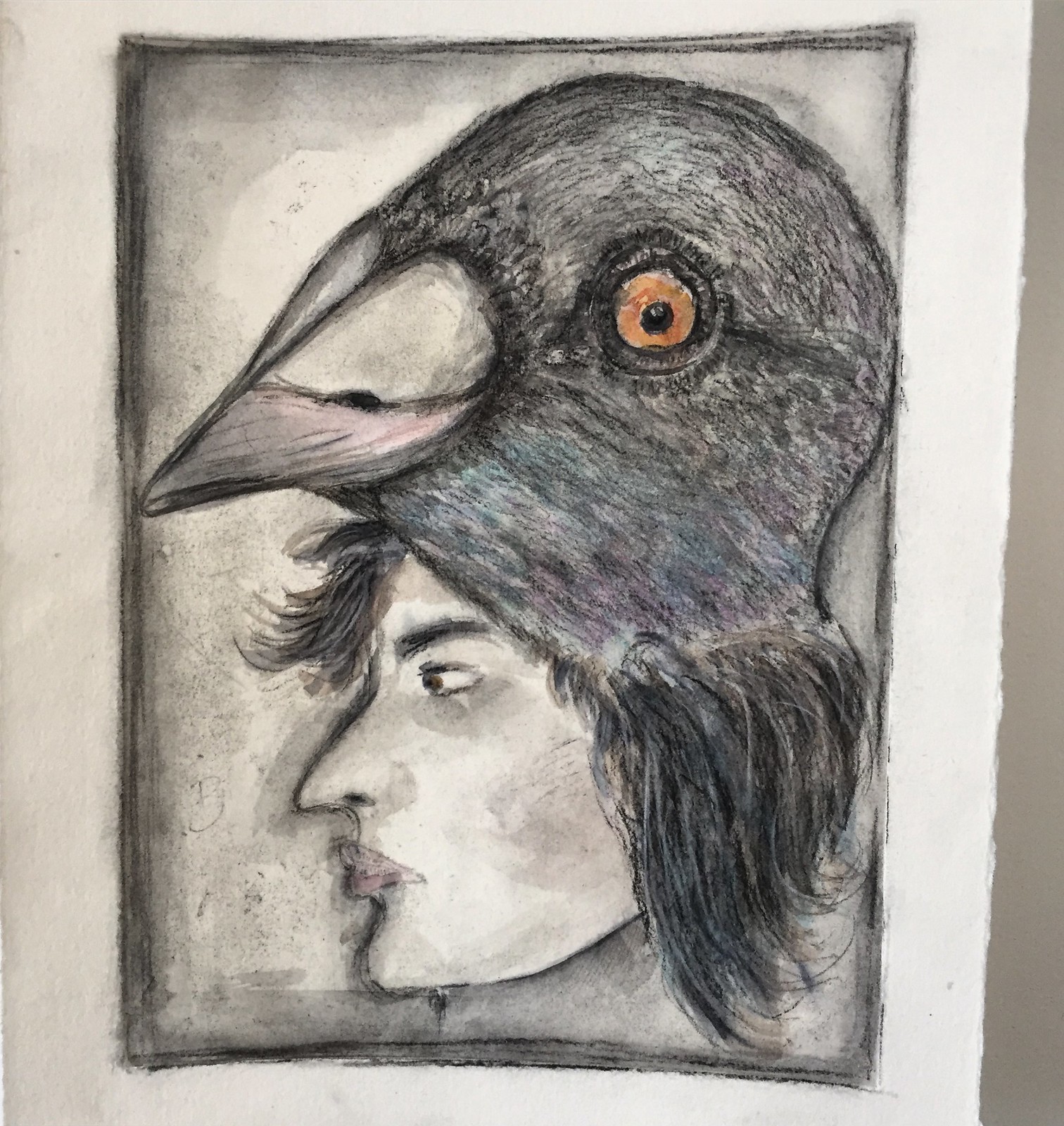This image portrays a detailed pen-and-ink drawing with charcoal-like shading on a piece of white paper. It features the profile of a woman's face looking to the left, illustrated with prominent lips, a large nose, and expressive features, all with light pink shading on the lips. Her dark hair flows down to shoulder length, spilling over her forehead and below her chin at the back. The background transitions from light to dark gray along the edges, with the drawing enclosed in a darker gray outline. The most striking element is the transition from the top of the woman's head to the head of a bird, depicted as though the bird's head is being worn as an oversized hat. The bird's head, shaded in dark gray, mirrors the size of the human head and features an orange eye with a black pupil. The beak, highlighted with a mix of gray and pink, completes the surreal fusion of human and bird elements in this portrait-oriented artwork.